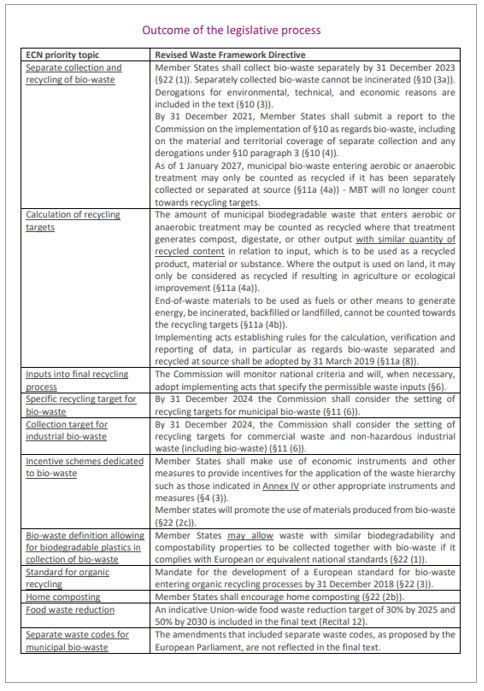**Detailed Caption:**

The image showcases a comprehensive document detailing the outcomes of the legislative process concerning the management and recycling of biowaste, set against a white background. At the top, the header "Outcome of the Legislative Process" is prominently displayed in purple text. Below this header, the main content is written in black text, delineating various sections regarding biowaste policies and practices.

1. **ECN Priority Topic: Separate Collection and Recycling of Biowaste**
   - **Revised Waste Framework Directive:**
     - Member states are mandated to collect biowaste separately by 31 December 2023.
     - Incineration of separately collected biowaste is prohibited.
     - Derogations for environmental, technical, and economic reasons are included.

2. **Reporting and Implementation:**
   - By 31 December 2021, member states must submit a report to the Commission on the biowaste collection implementation, covering material and territorial coverage, including any derogations under Article 10, paragraph 3.

3. **Recycling Requirements:**
   - From 1 January 2027, municipal biowaste entering aerobic or anaerobic treatment can only be counted as recycled if it has been separately collected or separated at the source.
   - Mechanical biological treatment (MBT) will no longer count toward recycling targets.

4. **Recycling Target Calculation:**
   - Municipal biodegradable waste entering aerobic or anaerobic treatment can be counted as recycled if it generates compost, digestate, or other similar outputs with recycled content used as products, materials, or substances.
   - Outputs used on land must result in agricultural or ecological improvement to be considered recycled.
   - Waste materials used as fuels, for energy generation, incineration, backfilling, or landfill cannot be counted toward recycling targets. Implementing acts establishing calculation, verification, and reporting rules for biowaste data shall be adopted by 31 March 2019.

5. **Inputs into Final Recycling Process:**
   - The Commission will monitor national criteria and may adopt implementing acts specifying permissible waste inputs.

6. **Specific Recycling Target for Biowaste:**
   - By 31 December 2024, the Commission will consider setting recycling targets for municipal biowaste.

7. **Collection Target for Industrial Biowaste:**
   - By 31 December 2024, the Commission will consider setting recycling targets for commercial and non-hazardous industrial waste, including biowaste.

8. **Incentive Schemes Dedicated to Biowaste:**
   - Member states are to use economic instruments and measures to incentivize the application of the waste hierarchy, promoting materials produced from biowaste.

9. **Biowaste Definition Allowing for Biodegradable Plastics:**
   - Member states may allow waste with similar biodegradability and compostability properties to be collected with biowaste if compliant with European or equivalent national standards.

10. **Standard for Organic Recycling:**
    - A mandate for developing European standards for biowaste entering organic recycling by 31 November 2018 is included.

11. **Home Composting:**
    - Member states are encouraged to promote home composting.

12. **Food Waste Reduction:**
    - The document includes an indicative union-wide food waste reduction target of 30% by 2025 and 50% by 2030.

13. **Separate Waste Codes for Municipal Biowaste:**
    - Proposed amendments for separate waste codes by the European Parliament are not reflected in the final text.